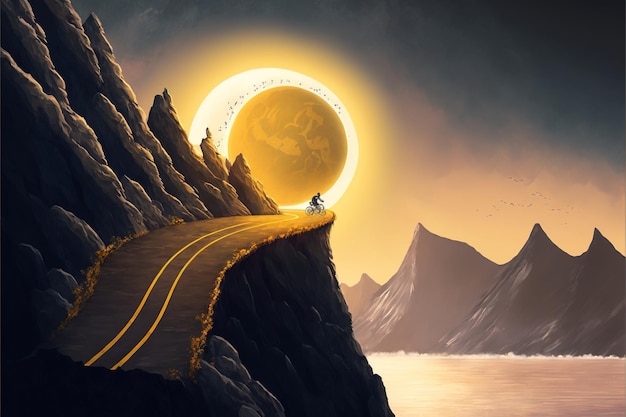The image is an animated depiction of a steep, winding road on the edge of a mountain cliff, bathed in the golden light of a massive sun, encircled by a prominent halo. The road, which features a double yellow line, leads up toward the seemingly colossal sun, creating a dramatic and somewhat surreal atmosphere. A tiny bicyclist is perched at the top part of the road, dwarfed by the immense size of the sun. To the right of the road, there are mountains and a body of water, over which a few black birds are flying. The sky in the background is a dark gray, contrasting sharply with the bright and clear natural lighting provided by the golden sun. The overall clarity and brightness of the animated scene highlight its otherworldly yet vivid nature.